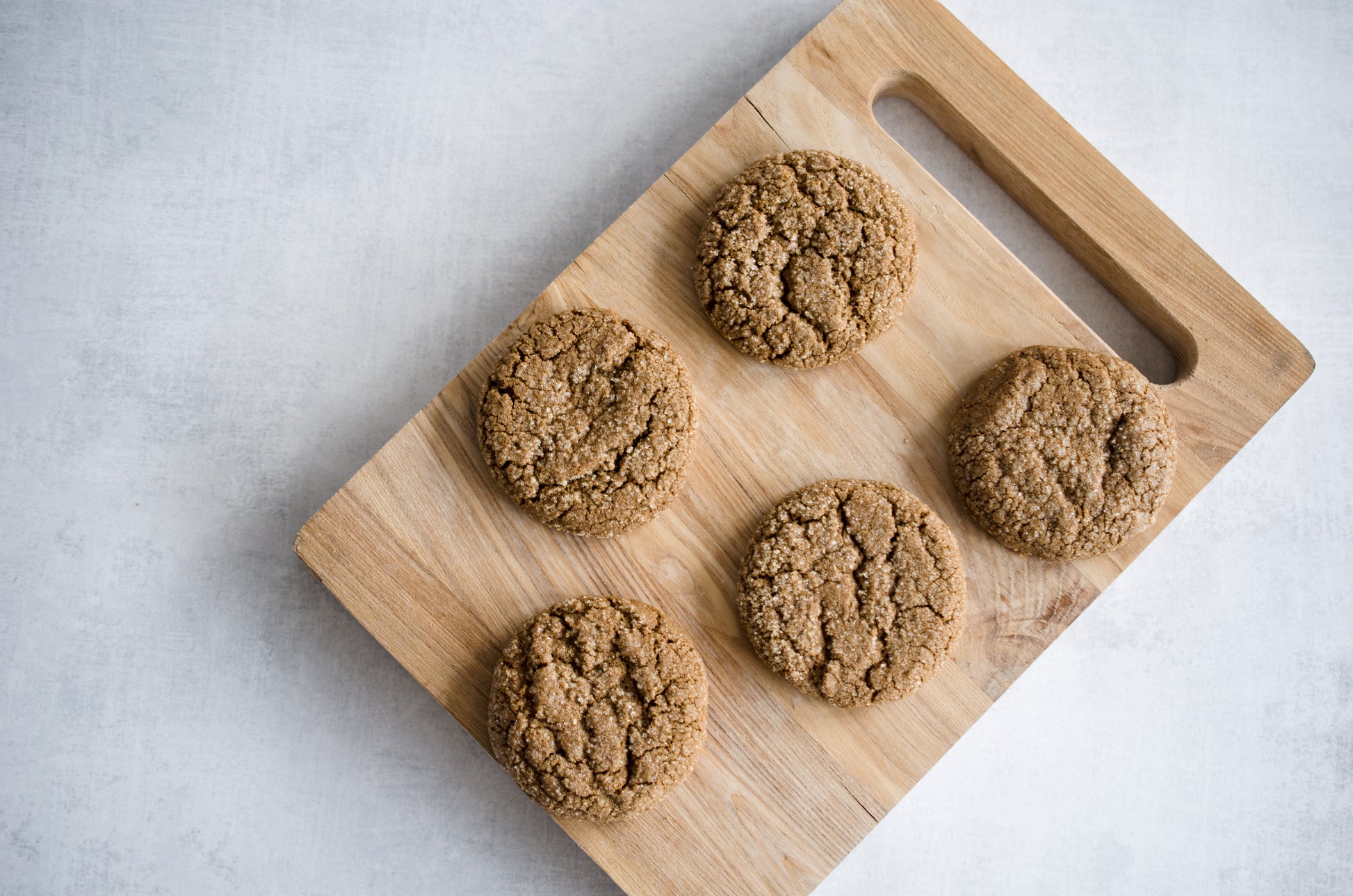This is a highly detailed overhead shot of five freshly baked cookies resting on a diagonally positioned cutting board. The cutting board, made of light to medium wood, features a long handle slot in the upper right-hand corner for ease of picking it up. The board also has a slight crack about an inch down from the slot. The cookies are brown, likely peanut butter cookies, sprinkled with granules of sugar and displaying little cracks indicative of their crunchy texture. They blend in with the board, both sharing a similar warm, brown hue. The background is a light to dark gray mottled surface, possibly a countertop, adding a muted contrast to the rich tones of the cookies and the cutting board.